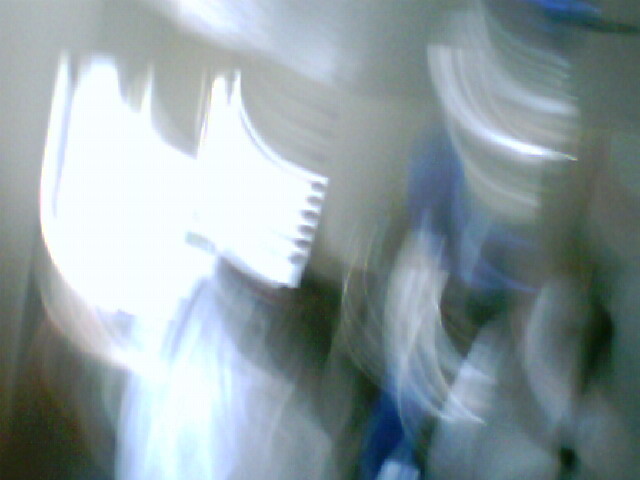The image depicts a surreal and abstract composition. At the top of the image, there are two white, curved shapes that resemble notebooks, though their exact nature is ambiguous. These shapes rest on a beige surface that features lined textures, adding an element of intrigue. Below the beige surface, a blue, curved form extends across the image, partially covering more white, curved objects. 

Towards the bottom of the scene, soft, puffy white shapes are visible, adding to the dreamlike quality. The image seems to be sideways, which contributes to the disorienting effect. Wisps of pink and blue hues intersperse throughout, with a particularly bright spot of light illuminating the left side. The entire composition has a brushed, wispy appearance, making it difficult to discern the definitive identity of each object.